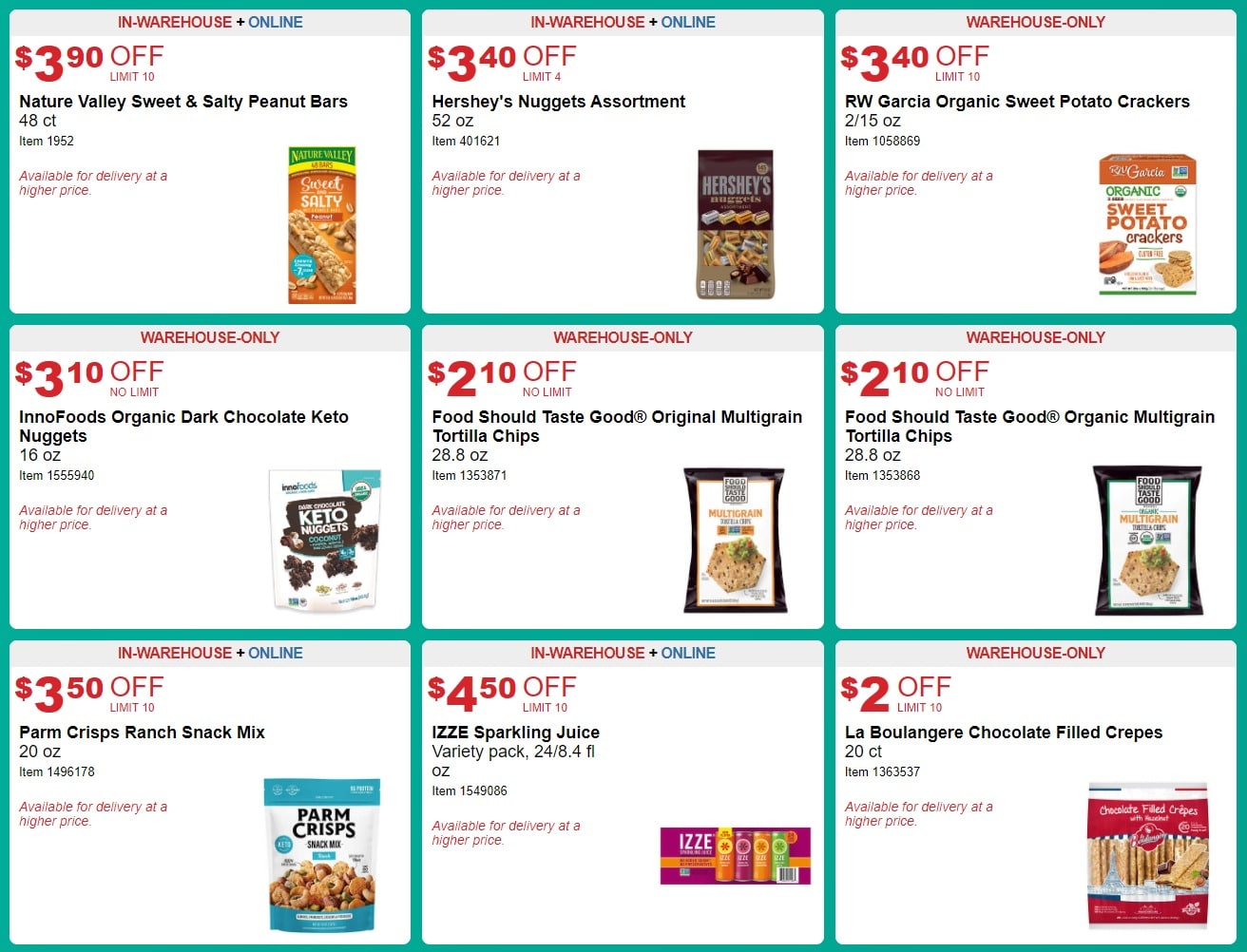In a bustling warehouse, vibrant blue lines delineate sections laden with Costco advertisements offering enticing deals. Among the standout bargains, shoppers can find $3.90 off on a 48-count pack of Nature Valley Sweet & Salty Nut bars. This offer is available both online and in-store, though delivery options might incur additional charges.

An array of discounted items includes the Hershey's variety, with notable savings of $2.40 off, and RW Garcia's organic sweet potato crackers, marked down by $3.10 with no purchase limits. These crackers, item number 1058869, come in boxes amid stacks of other organic and keto-friendly snacks. For instance, the Nature's Food Organic Dark Chocolate Keto Nuggets, item 155940, are available at $2.10 off their usual higher price.

Other tempting deals include Food Should Taste Good's organic multi-grain tortilla chips, item 135, offered at an attractive discount. Shoppers can also take advantage of a $4.50 reduction on the Sparkling Juice Variety Pack, containing twenty-four 8.4 fluid ounce bottles, item 1549086.

The warehouse aisle also features a selection of chocolate-filled crepes, nestled among the myriad of health-conscious and indulgent treats—each item meticulously listed and marked for conscientious shoppers seeking both value and quality.